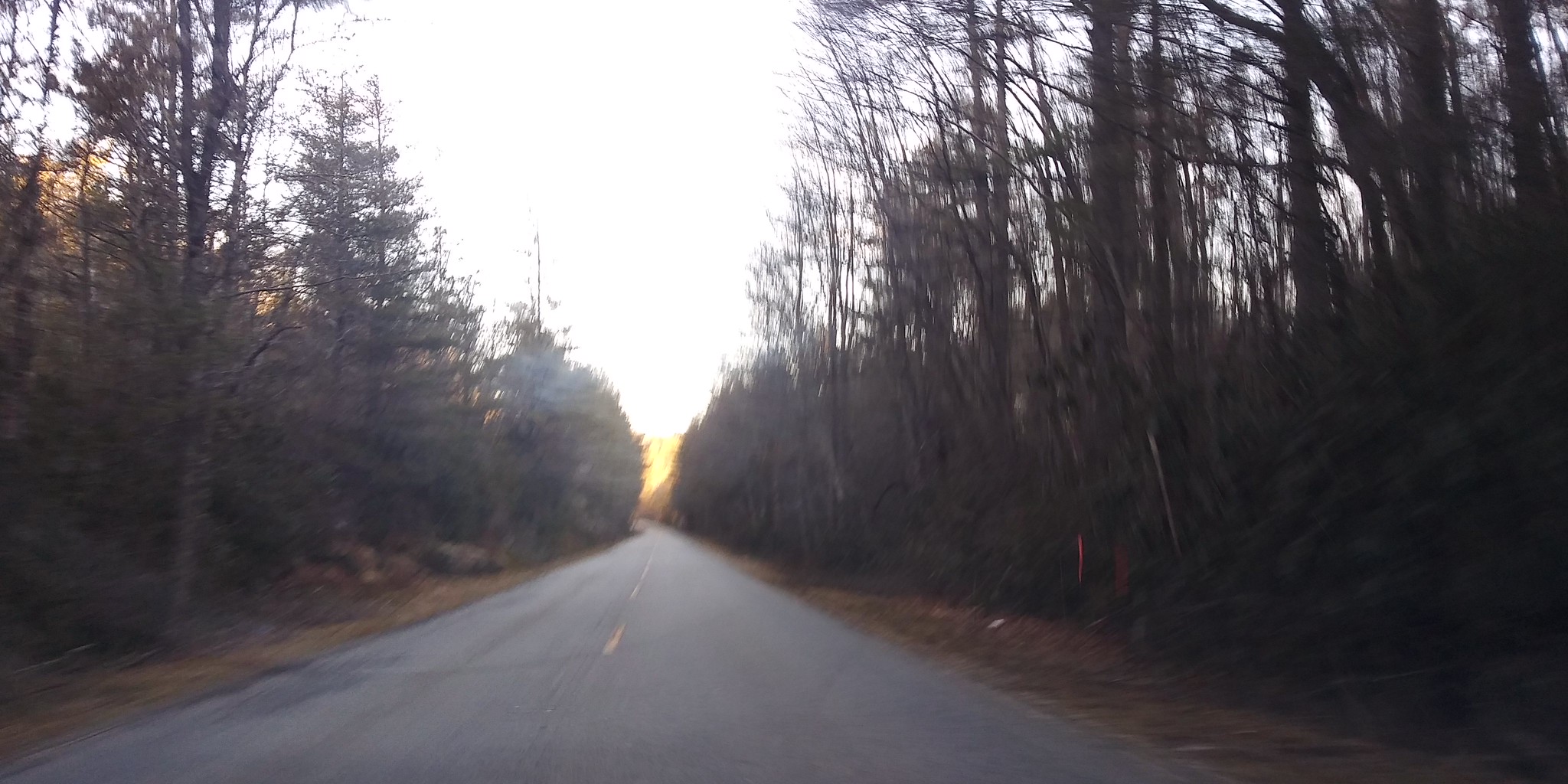The outdoor color photograph captures a two-lane road, marked by a yellow dashed line, curving slightly to the left as it extends from the foreground into the distance. The scene is illuminated by bright daylight, possibly during sunrise or sunset, casting shadows on the subject. On the left side of the road, tall evergreen trees about two stories high are visible, while on the right, taller deciduous trees, their trunks standing around two and a half to three stories tall, dominate the view. Despite some foliage remaining on the left-side trees, most of the right-side trees appear barren, suggesting the photo was taken in late fall or winter. The sky is clear and white, with a hint of sunlight peeking through in the distant background. The image conveys a sense of isolation as there are no other vehicles on the road, and while it is well-lit, it remains slightly out of focus.